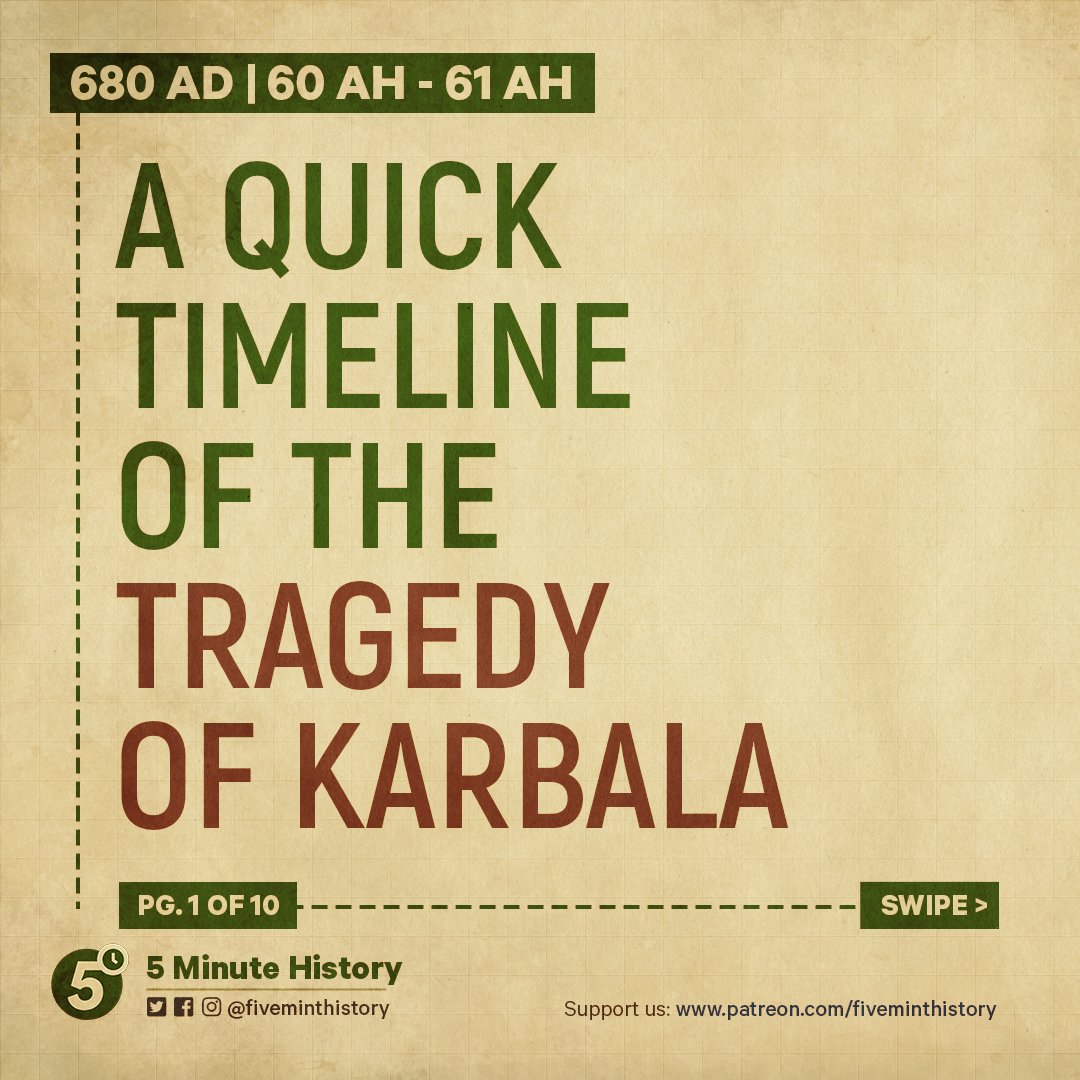The infographic features a detailed timeline of the Tragedy of Karbala, framed within a beige or tan background. At the top left corner, within a black bar and white lettering, it reads "680 AD / 60 AH - 61 AH". Below this, in larger text with "A Quick Timeline of the" in green and "Tragedy of Karbala" in dark maroon, the title stands out prominently. A green dotted line vertically traverses the left side from top to bottom.

At the bottom of the infographic, a black bar states "Page 1 of 10" in white text and another section advises to "Swipe" along a dotted line leading to the right. The bottom left corner features a logo with a green circle encompassing the number "5," accompanied by "5-Minute History." Additional text encourages support through "www.patreon.com/5-MinHistory," and social media handles, including "@5-MinHistory" on Twitter and Facebook, emphasize engagement.

The careful use of green and maroon text highlights key information, while the structured layout ensures clarity and ease of navigation.